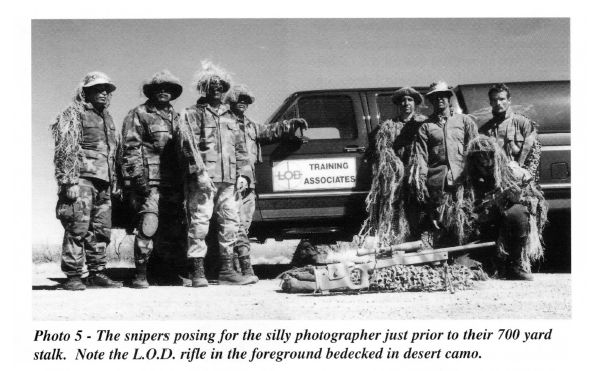This black and white photograph features eight military men dressed in camouflage outfits, most wearing hats with wide brims and some adorned with grass atop. They are arranged in two symmetrical groups: four on the left side and four on the right side, with one man kneeling. The group is posed in front of a dark pickup truck which has a canopy on the back and a white sign on the driver's door reading "LOD Training Associates," accompanied by a sniper symbol. The setting appears to be a barren, dirt landscape under an open sky, which adds to the starkness of the image. The cumulative focus of the photograph is not just on the men but also on a prominent sniper rifle in desert camo, positioned in front of the group to the right, lying on some sort of mesh material. The bottom of the image features a strip of white with black italicized text that reads: "Photo 5 – The snipers posing for the silly photographer just prior to their 700-yard stalk. Note the LOD rifle in the foreground bedecked in desert camo." The composition and details suggest the image might be from a historical or military publication.